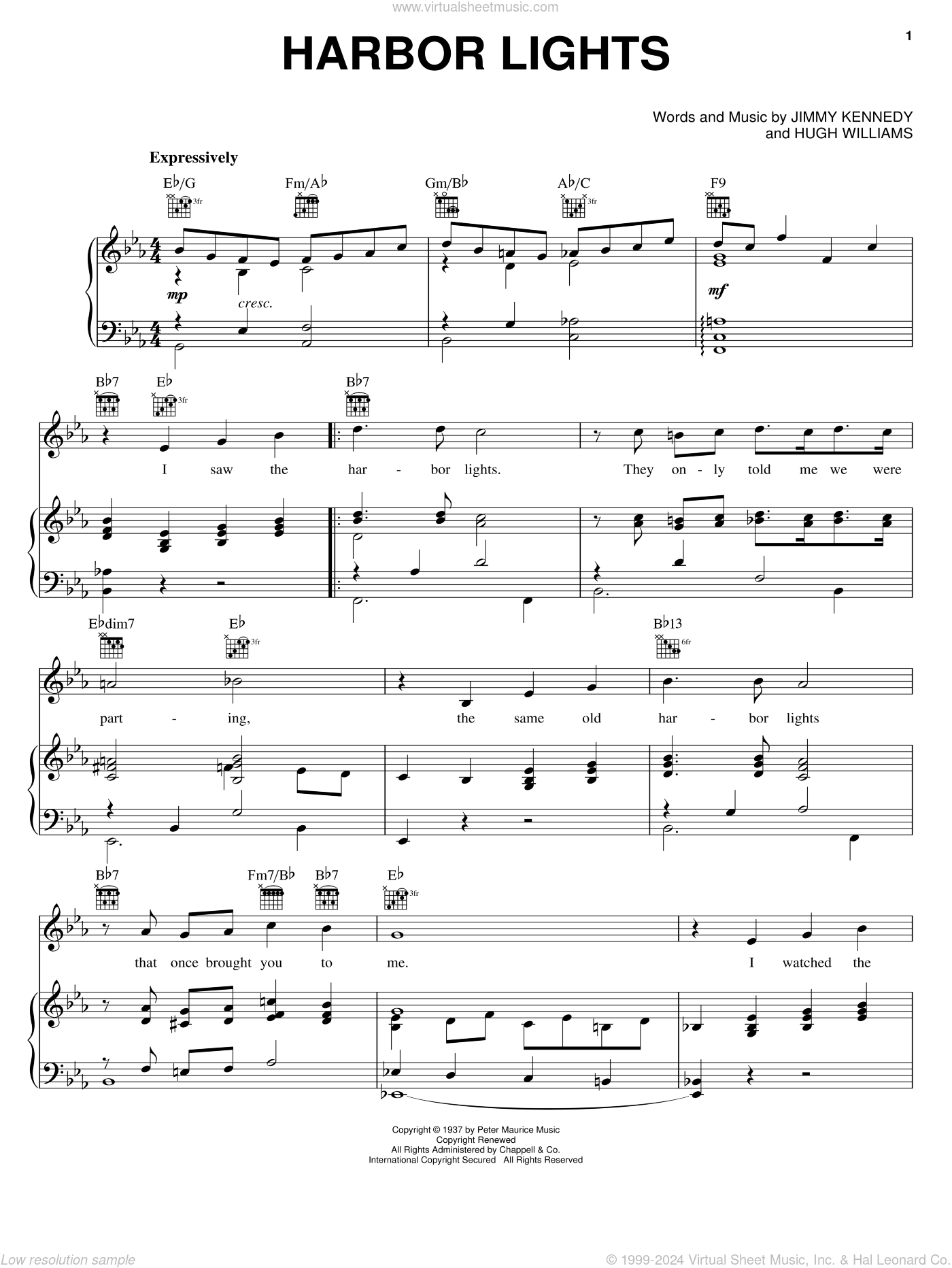The image depicts a vertically rectangular piece of black and white sheet music against a plain white background. At the top, in very small light gray text, it reads "www.virtualsheetmusic.com." Below that, in large black capital letters centered on the page, it says "HARBOR LIGHTS." Further down and slightly to the right, in smaller print, it says "WORDS AND MUSIC by Jimmy Kennedy and Hugh Williams." The sheet contains eight lines of music with both treble and bass clefs, suggesting a possible combination of voice and piano parts. The first chord notated is E flat/G, followed by F minor, A flat, G minor, B flat, A flat/C, and F 9 in succession. Expressively is indicated in bold on the left side near the music annotations. At the bottom of the sheet, centered, is the copyright information, stating "Copyright 1999 to 2021 Virtual Sheet Music Inc and Hal Leonard Co." with additional low-resolution sample text on the lower left.